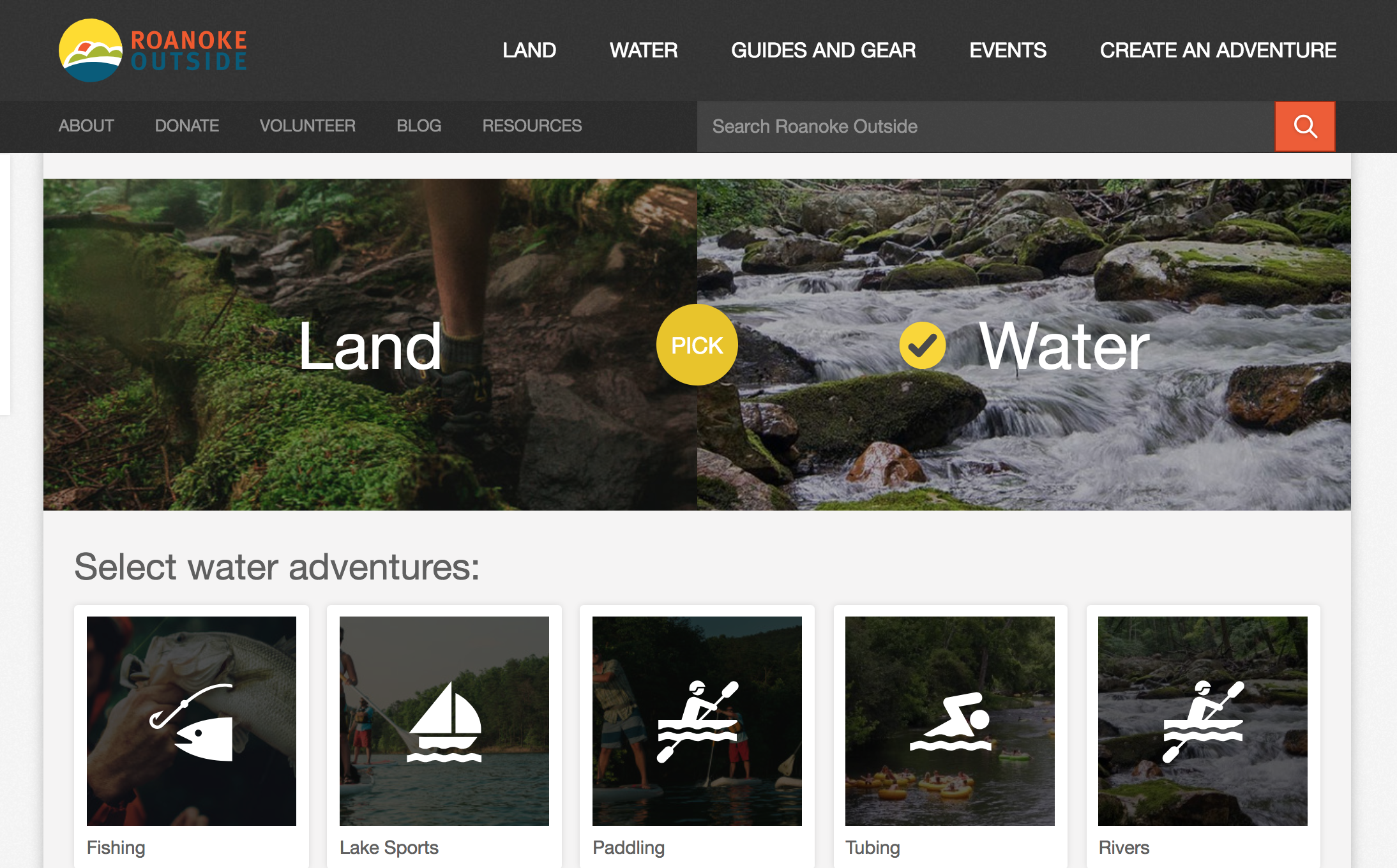The screenshot appears to be from a website dedicated to outdoor adventures. In the top left corner, there is a logo with the text "Roanoke Outside." To the right of the logo, there is a menu bar featuring the options: "Land," "Water," "Guides & Gear," "Events," and "Create an Adventure." The menu is displayed on a black background with white text for easy readability.

Beneath this primary menu, there is another navigation bar, also on a dark black background, but with grey text. This secondary menu includes options such as "About," "Donate," "Volunteer," "Blog," "Resources," and a search bar positioned to the right.

The main section of the page has a split theme, offering users a choice between "Land" and "Water" adventures. The left side features an image representing land-based activities, while the right side showcases water-based activities. In this particular screenshot, the water activities option appears to have been selected, as indicated by a highlighted state.

Below this selection section, there is a category titled "Select Water Adventures." This category offers several sub-options: "Fishing," "Lake Sports," "Paddling," "Tubing," and "Rivers." Each sub-option includes a real photograph in the background, overlaid with a white graphic representative of the activity. For instance, the fishing option has an image of a fish with a fish graphic on top of it.